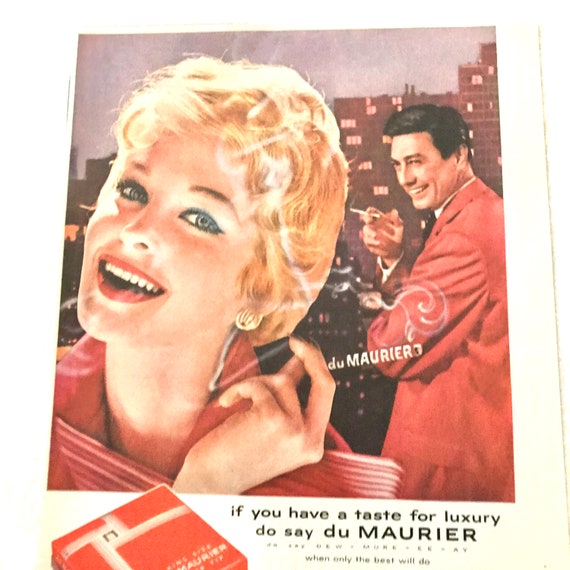This vintage cigarette advertisement, likely from the 1950s or 1960s, features a meticulously illustrated scene set against a city backdrop with softly lit buildings under a gray sky. In the foreground, a smiling blonde woman with short hair and blue eyes captures attention as she gazes directly at the viewer, a gold earring dangling from her ear. Her cigarette, emitting a delicate curl of smoke, prominently displays the brand name, Du Maurier. To the right and slightly behind her, a man with dark hair dressed in a red suit looks towards her with a smile, also holding a cigarette. Both figures are enveloped in a luxurious ambiance, augmented by the elegant, retro attire they wear. At the bottom of the image, a packet of Du Maurier cigarettes sits beside bold text proclaiming, "If you have a taste for luxury, do say Du Maurier. When only the best will do." This ad epitomizes an era when sophistication and elegance were seamlessly tied to the act of smoking.